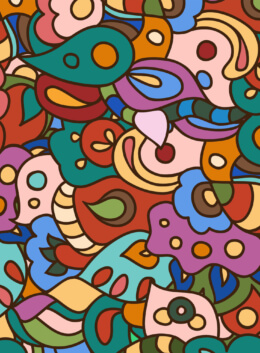This digital illustration features a vibrant medley of overlapping shapes and colors, epitomizing abstract art through its meticulous use of clean lines and flat color sections. It is a portrait-style composition filled with paisley, floral, teardrop, leaf, and ribbon shapes, as well as amorphous and cloud-like forms. The shapes are outlined in black, creating a stark contrast that accentuates each element. The artwork boasts an eclectic palette that includes hues of red, green, teal, purple, orange, pink, blue, and light shades of yellow and beige. Various shapes, from symmetrical dots to elongated tubular forms with yellow and gold striping, intermingle in a harmonious yet random fashion, covering the entire canvas with no consistent border, making the illustration a vivid expression of imaginative digital media.